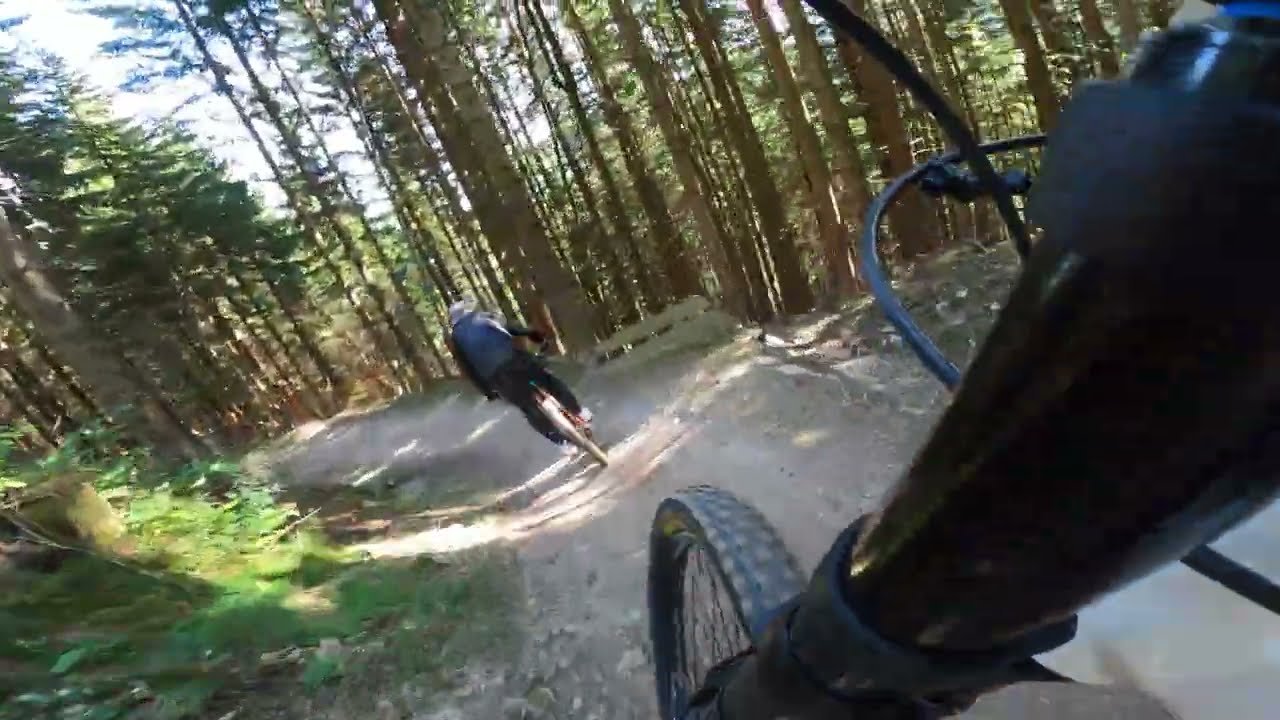The photograph, captured from the perspective of a camera mounted on the front fork of a mountain bike, offers a thrilling view down a steep, curved mountain trail within a dense grove of tall, thin pine trees. The scene is illuminated by bright daytime sunlight, filtering through the foliage. In the foreground, the bike's knobby front tire, brake cables, and shift levers are visible, emphasizing the rider's focus on the rugged path ahead. Down the trail, another cyclist, dressed in black pants, a dark coat, and white athletic shoes with a crusher-type hat, navigates a left curve towards a slight fence on the right. The trail itself is dusty gray, bordered by a hillside interspersed with rocks, grass, and a logged tree stump, creating a dynamic and immersive depiction of mountain biking through scenic wilderness.